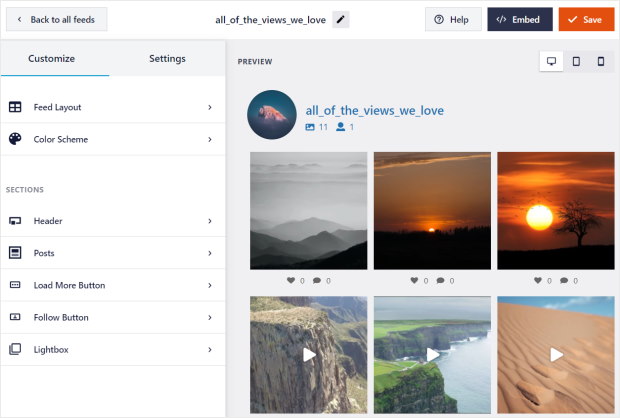A breathtaking gallery showcases the beauty of nature through a series of stunning images. The first photograph is a striking black-and-white capture of majestic mountains under a vast sky, evoking a sense of timeless grandeur. Following this, a vivid shot of a sunset reveals the horizon ablaze with rich hues of orange and gold, as the sun serenely descends behind the landscape. The third image captures the sun in its full glory, nestled beside a solitary tree, with the sky gradient transitioning from yellow to deep orange, creating a mesmerizing contrast. The fourth image features a rugged cliff, inviting viewers to explore further with clickable arrows that hint at video content. Next, a lush, green cliff reminiscent of the verdant landscapes of Bermuda captivates with its vibrant colors. The penultimate image is a serene portrayal of a vast sand dune, its surface elegantly patterned by the wind's gentle embrace. Toward the left, user interface options for customization, settings, and layout adjustments are conveniently displayed, offering a tailored viewing experience.